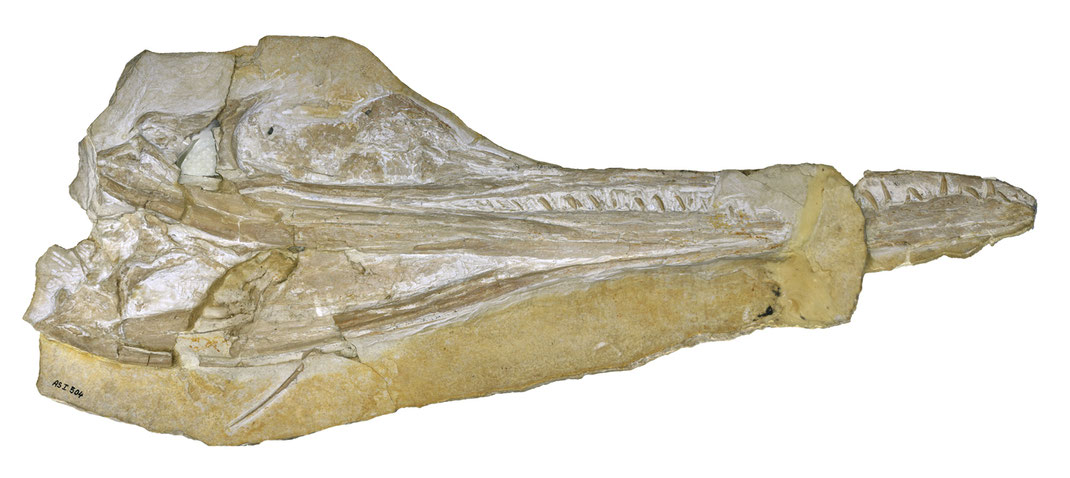In this detailed photograph, we have a centrally located stone object, lying horizontally on its side against a completely white background. The object is captured in a close-up manner revealing its texture and intricate details. It appears to be a fossil or a rock formation, possibly part of a bone structure suggesting it could be from a museum's educational collection. The colors seen are varying shades of white, tan, black, and gray, with white veins adding to its texture. The object displays distinct grooves, suggesting a rough surface overall, while the edges appear smoother. Notably, there are up-and-down notches along the central spine-like feature of the rock, resembling the vertebrae of a backbone. Additionally, the rock formation narrows towards the center and then appears to end or perhaps transform into a round area before narrowing further, almost resembling a lizard's head. Handwritten letters and numbers, possibly "ASI B04", are faintly visible in the far left-hand corner at the bottom of the stone, though they are not clearly legible.